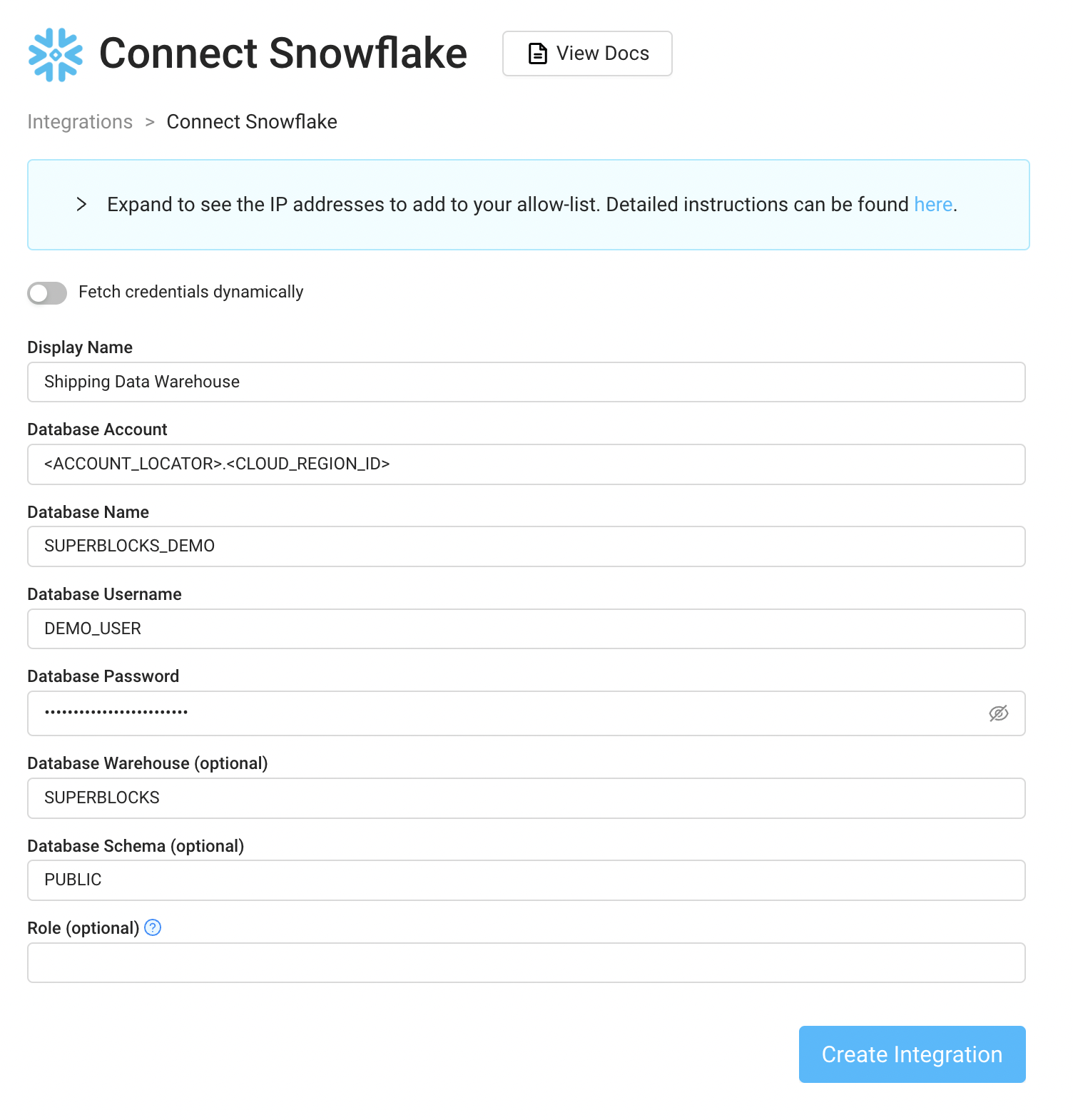The image depicts a section of a web page titled "Connect Snowflake." At the top, there is an option labeled "View Docs" located beside the main title. Below, an area titled "Integrations" features an arrow pointing to "Connect Snowflake." 

Just underneath this section, a teal-colored box instructs users to "expand to see the IP addresses to add to your allow list," with a note that detailed instructions can be found via a hyperlink, which is in blue.

Further down, there is a toggle switch labeled "Fetch credentials dynamically," which is currently in the off position with the slider ball towards the left. Additional fields include "Display Name" with an example entry "shipping data warehouse," followed by "Database Accounts" which lists fields like "account_locator," "cloud_region_id," "database name," "database username," "database password," and "database warehouse." Certain fields like "database schema" and "role" are marked as optional.

In the lower right corner of the interface, a blue button labeled "Create Integration" is visible, prompting the user to proceed with the integration setup.